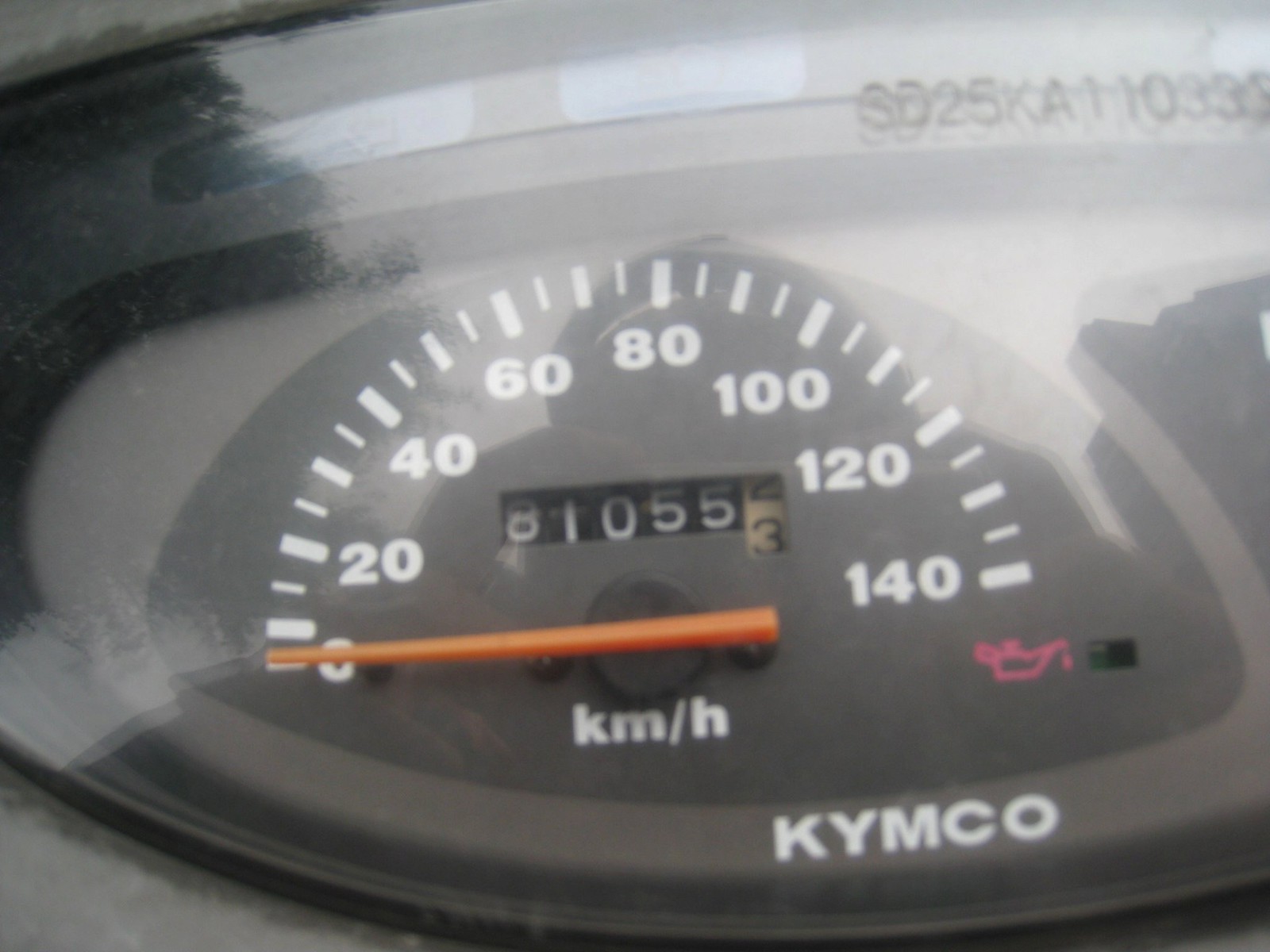The image features a close-up shot of a car speedometer, encased behind a reflective glass or plexiglass surface. Central to the image is the speedometer itself, calibrated in kilometers per hour and marked from zero up to 140 km/h. Underneath the 140 km/h marking, there is a small oil can icon that serves as a reminder for oil changes. The odometer within the speedometer displays a reading of 81,055 kilometers, with the needle pointing just past the 80,000 km mark.

To the left and right of the speedometer are various indicators, including what appear to be blinkers for left and right turns. The bottom right section of the speedometer area features the brand name "Kymco," spelled out in capital letters. In the top right corner, a serial number or VIN is faintly visible, though it is not clear if this is on the glass or a reflection on its surface. Subtle reflections, including that of the individual taking the picture, add another layer to the image. Blue indicators above the main display suggest additional sensors or warning lights.